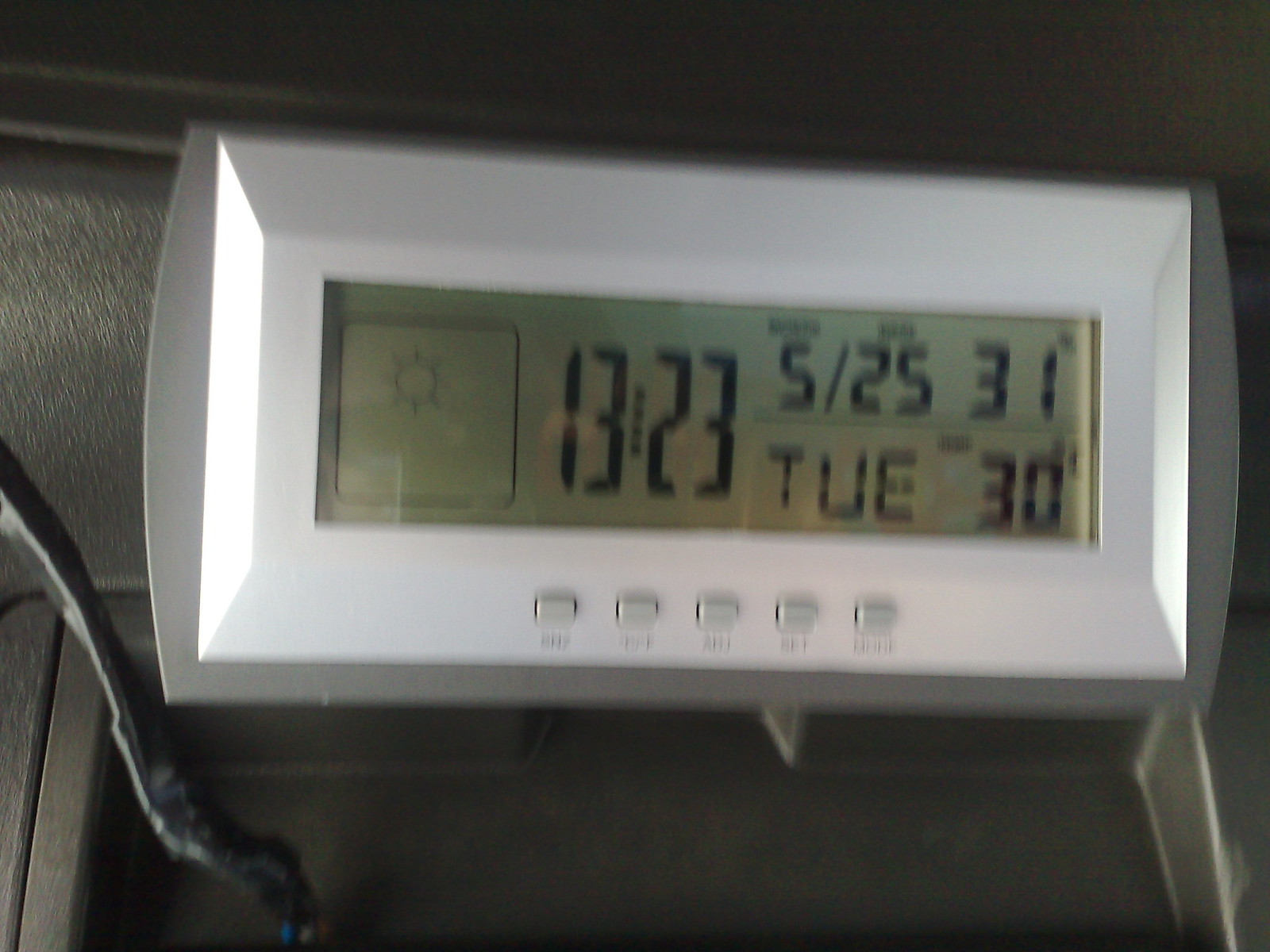The image showcases a piece of equipment featuring a digital display. The display, shaped as a white rectangle, has an olive green background. On the left side of the display sits a square with a faint gray drawing of a sun. Adjacent to this square, the number "13" is displayed, followed by vertical lines, and then the number "23," which likely represents the time in military format. 

To the right of these numbers, there are two rows of additional information. The top row shows the month and day, denoted as "525," while the number "31" is displayed alongside. Beneath that, the bottom row reads "Tuesday" and the number "30." Situated below the digital display are several small, rectangular raised buttons, allowing interaction with the equipment.